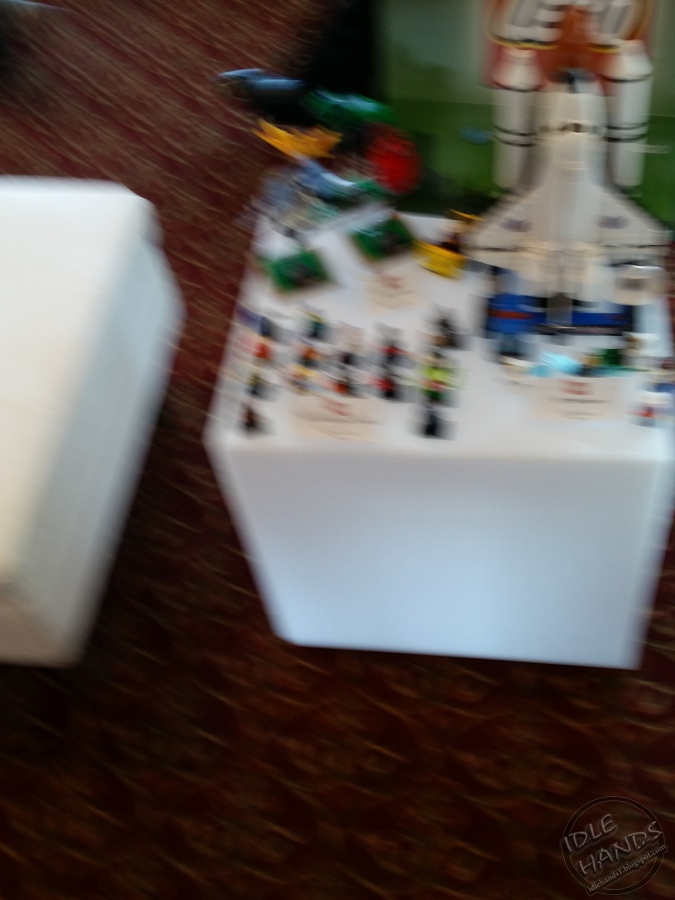In this blurred image, a scene unfolds on a dark wine-colored carpet adorned with a gold design. Central to the composition is a white block table partly accompanied by what seems to be a white ottoman or reclining chair. Dominating the tabletop is a detailed NASA space shuttle, featuring distinctive white and black striping, possibly modeling the Columbia. To the left and surrounding the shuttle are various colorful Lego pieces, with specific hues like black, orange, red, and green, alongside small figurines that resemble Lego men. The background is marked by the word "Lego" in red and white letters, likely printed on a box. Two white cubes, possibly ottomans, are partially visible, one of which holds part of the Lego arrangement. Adding a final touch, the phrase "idle hands" is subtly inscribed in white at the bottom right corner of the image.